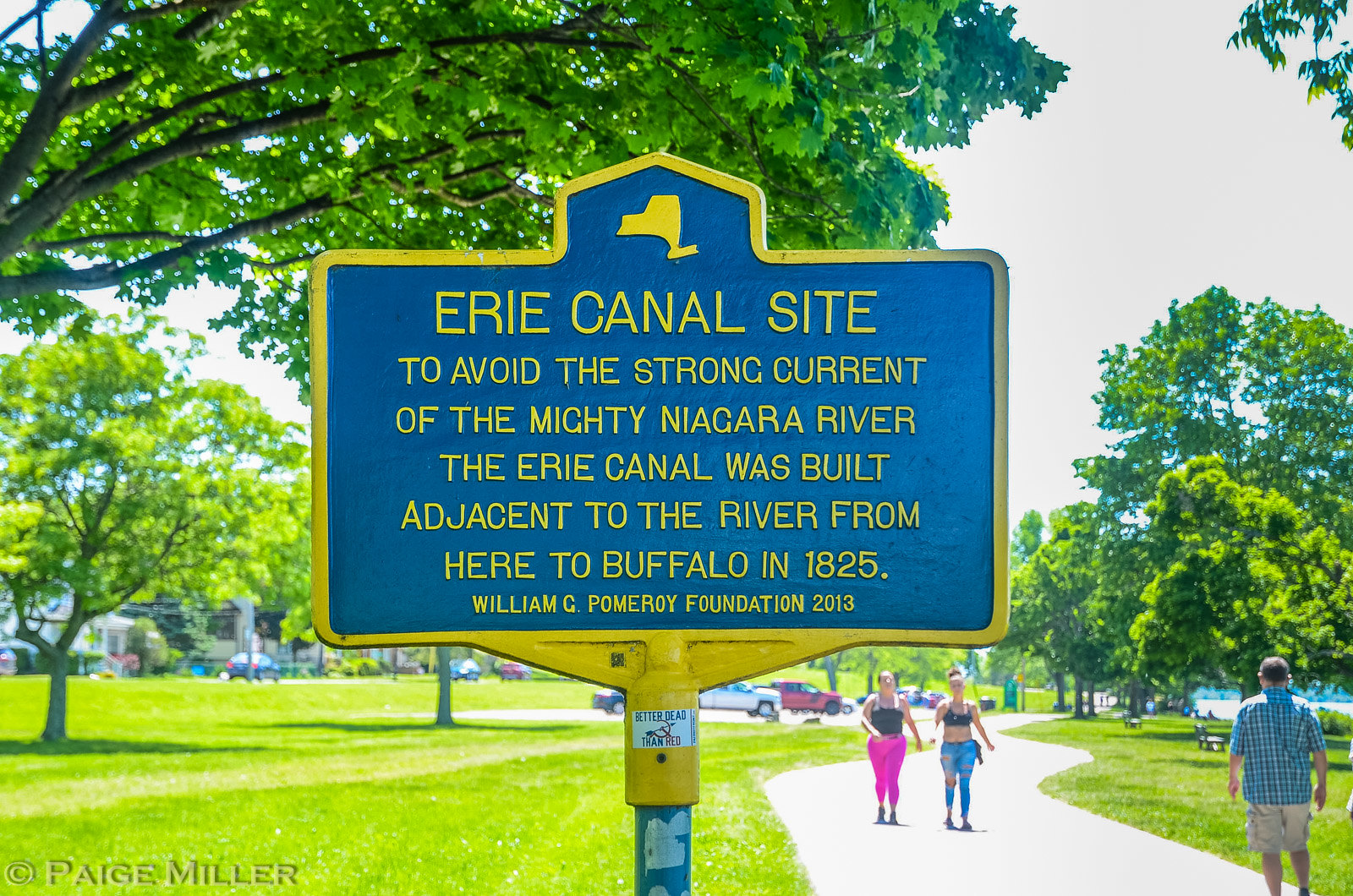The image captures a historical sign about the Erie Canal, prominently placed in the center on a metal post. The rectangular sign features a distinct pointed top and is framed with a yellow border. The background of the sign is a deep blue, filled with yellow text detailing its significance. An illustration of the state of New York can be seen at the top of the sign. The sign reads, "Erie Canal site to avoid the strong current of the mighty Niagara River. The Erie Canal was built adjacent to the river from here to Buffalo in 1825. William G. Pomeroy Foundation, 2013."

Surrounding the sign is a lush environment with expansive green grass and towering trees with full, green leaves. A concrete walkway runs along the right side of the image, where three people are strolling—one man and two women, possibly in workout or casual attire. In the distant background, additional elements like picnic tables, cars parked and moving, and possibly a parking lot enhance the park-like setting. The picturesque setting suggests the sign is located in, or near, a state park, reflecting both natural beauty and historical significance.